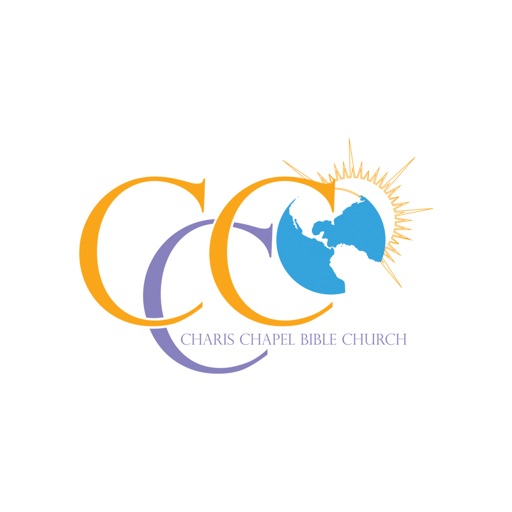The logo for the religious institution features a white background with three overlapping 'C's arranged in a distinctive manner. The first 'C' is orange and located at the left-hand side. Slightly below and to the right of it, there is a second 'C' in purple. The third 'C' is orange again and sits to the right of the purple 'C', aligning at the same height as the first 'C'. At the center of these 'C's is a globe, showcasing the landmasses in white and the water in a vibrant blue. Behind the globe, there's an image of the sun, characterized by its spiky, yellow rays extending outward, suggesting the warmth and brightness of sunlight. Wrapping inside the curvature of the second 'C' in purple font at the bottom, the text "CHERISH CHAPEL BIBLE CHURCH" appears in all capital letters, also in a purple hue, completing the emblem of this religious institution.